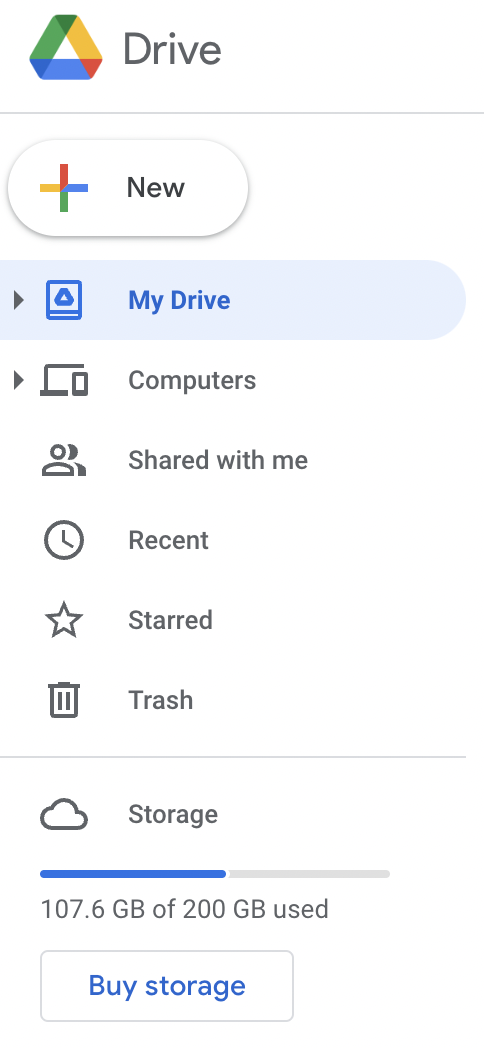The Google Drive interface is depicted with its characteristic triangular logo featuring specific color sections: green at the top left, yellow at the top center, red at the bottom right, and blue at the bottom left. The interface displays the following sections: "My Drive," "Computers," and "Shared with me." Icons representing a laptop and a phone appear under the "Computers" section, indicating a connection to these devices. The "Shared with me" section includes an icon of a person alongside a clock symbol for the "Recent" section. Additionally, the "Trash" section is highlighted, which appears to contain numerous items. The storage information indicates that 107.6 GB out of 200 GB are used. The background of the interface is white, with various options available for managing files and storage. There is also a prominent rectangular area displaying storage information.